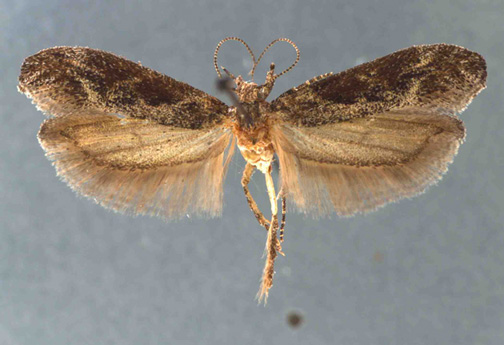In this detailed photographic image, set against a textured gray background with varying shades and a small black spot near the bottom middle section, a moth is prominently displayed facing the camera and slightly upward. The moth has four wings: the upper two are dark brown with brown spots, while the lower two are lighter brown with a fringed edge. Four of the moth's legs are visible extending from underneath its body, and its antennae are also clearly visible, intriguingly folded in a way that shapes a heart design. Despite the natural appearance, it appears the moth is either dead or being held in place, possibly suspended by a string or a pin, adding an interesting element to this unique capture. The out-of-focus background enhances the sharp details of the moth, spotlighting its intricate features.